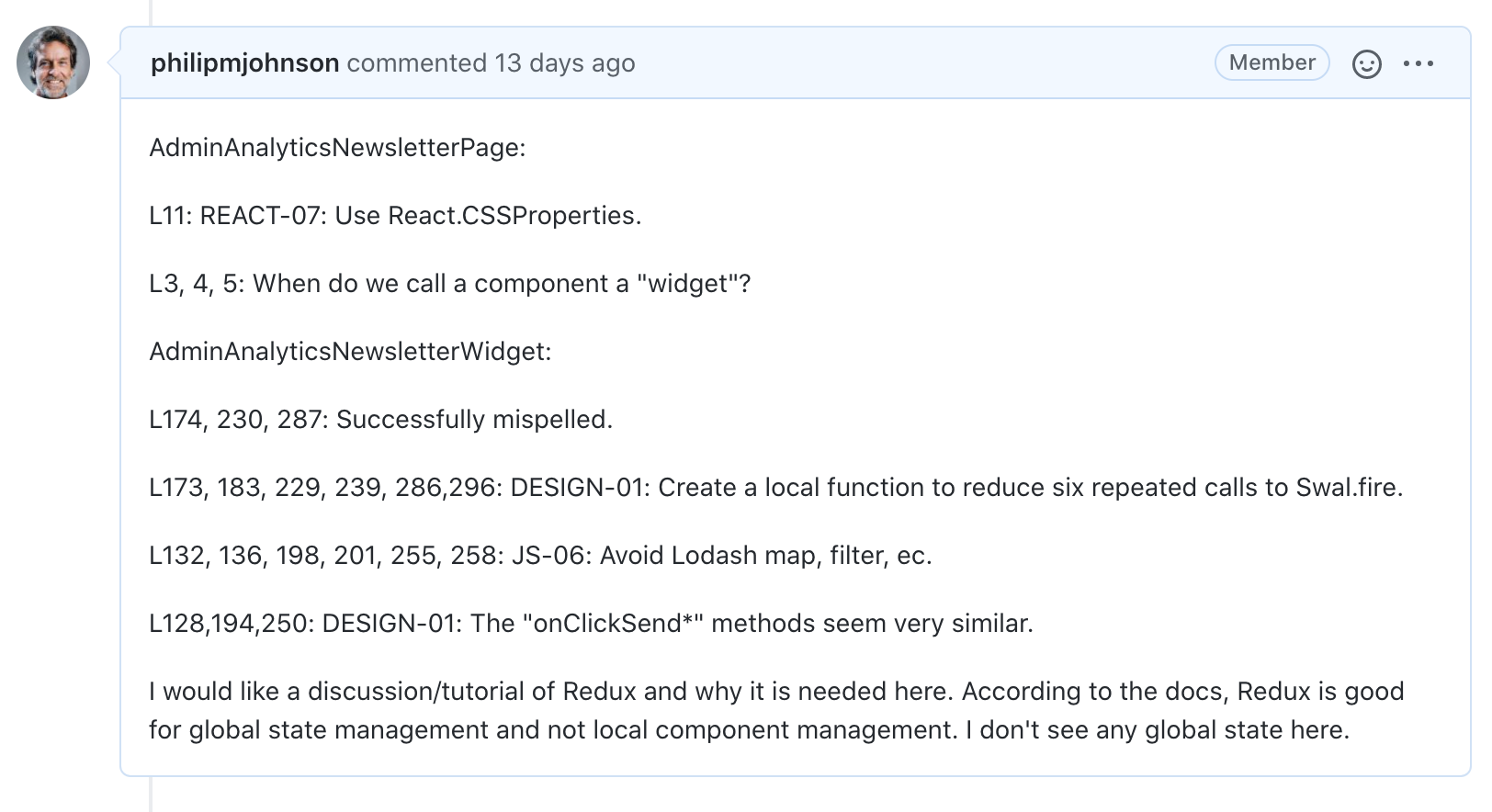The image displays a detailed snapshot of a comment or chat thread on an online platform. The comment is authored by Philip M. Johnson, whose name and small profile picture are prominently displayed at the top of the comment box. The comment was posted 13 days ago, indicating its recent relevance. Philip appears to be an active member or account holder on this particular website.

In his comment, Philip contributes intriguing points involving admin analytics and a newsletter page. The comment lists several entries preceded by the letter "L," such as L11, L345, L174, and L230, among others. Beneath these entries, Philip writes a thoughtful statement requesting a discussion tutorial on Redox and its necessity on the platform. He specifically notes from the documentation that Redox is beneficial for global state management but not for local management, expressing his confusion due to the absence of global state in the current context.

It is evident that Philip is seeking to address a concern or clarify a concept related to Redox, perhaps to better understand its application or resolve an issue. The detailed comment reflects a user engaged in a critical analysis, aiming to improve his comprehension or the functionality of the discussed topic.